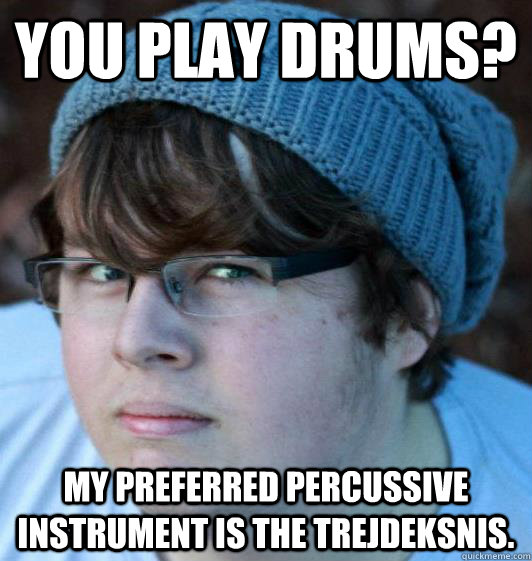The image depicts a shirtless, bald, and muscular white man with a goatee and mustache, crouched on all fours on a bed. He has a stern look on his face and sports a tattoo of Darth Vader's head near his upper right shoulder. A belt with a strap that goes underneath his buttocks is visible. The bed features a brown headboard and tall bedposts against a dark-colored, possibly grainy cement or brick wall. The bedspread is a camouflage pattern in red, gray, black, and white, complemented by black sheets and pillows with white stripes. White text overlay near the man's body reads "HI-H-A-I." Two white electrical outlets are visible at the bottom corners of the image.